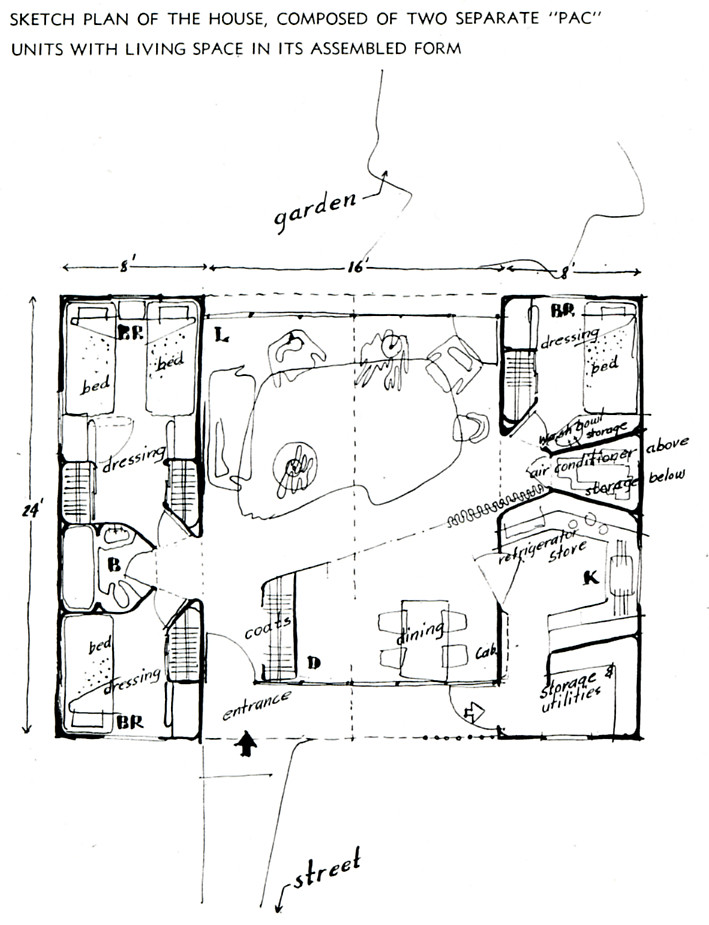This is a detailed illustration rendered in black pen, resembling a hybrid of a blueprint and a sketch. At the top, it is labeled "Sketch plan of the house composed of two separate PAC units with living space in its assembled form." The floor plan showcases a rectangular house with designated living spaces and annotations for easy identification. The entrance is marked with an arrow pointing to the street, and a garden is indicated in the back.

The house features various rooms marked with specific labels. The living room (L), dining room (D), bedroom (BR), bath (B), and kitchen (K) areas are clearly designated. The dining room is centrally located with a dining table, and the living room contains chairs and a sofa. On the left side of the sketch, there is a small bedroom with two beds and a dressing area adjacent to a bathroom. Another bedroom with a single bed is situated at the bottom, while a third bedroom occupies the top right corner.

The air conditioning unit is positioned along the right wall, adjacent to the kitchen, which includes a refrigerator and a stove. There is also a note mentioning "air conditioner above" and "garage below." The drawing includes measurements, showing dimensions of 24 inches in height and 16 by 8 inches in length. Additionally, the plan highlights storage areas, a utility room, and a closet for coats. The overall layout provides a comprehensive view of the organized and functional space within the house.